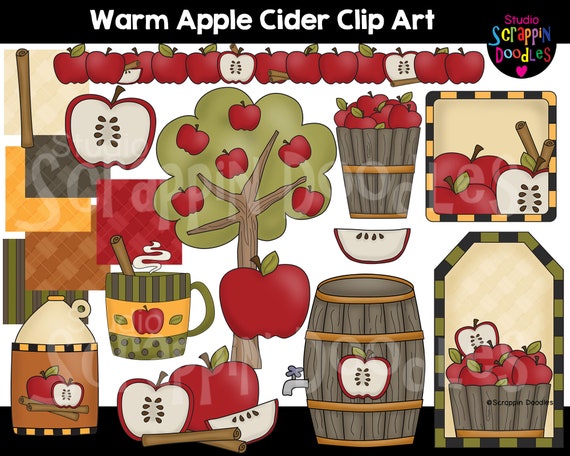This horizontally oriented, hand-drawn or computer-animated graphic is a vibrant and cartoony display celebrating various uses and depictions of red apples and apple cider. The illustration, titled "Warm Apple Cider Clip Art" at the top, is adorned with fall colors—reds, browns, oranges, and yellows—against a white background and framed by black borders at the top and bottom. 

In the image, an apple tree laden with red apples stands out, set alongside barrels brimming with apples and apple cider, one of which features a spigot. There are also sliced apples showcasing their seeds, and a ceramic cup with apple slices and cinnamon sticks implying a hot apple cider drink. Additionally, there are jugs of apple cider scattered throughout the scene. The bottom right features another barrel filled with a mix of whole and sliced apples. A tag in the top right corner reads "Studio Scrapping Doodles," suggesting the artist's signature or the collection's name. This detailed, decorative graphic captures the essence of apples and apple cider in a cozy, autumn-themed presentation.